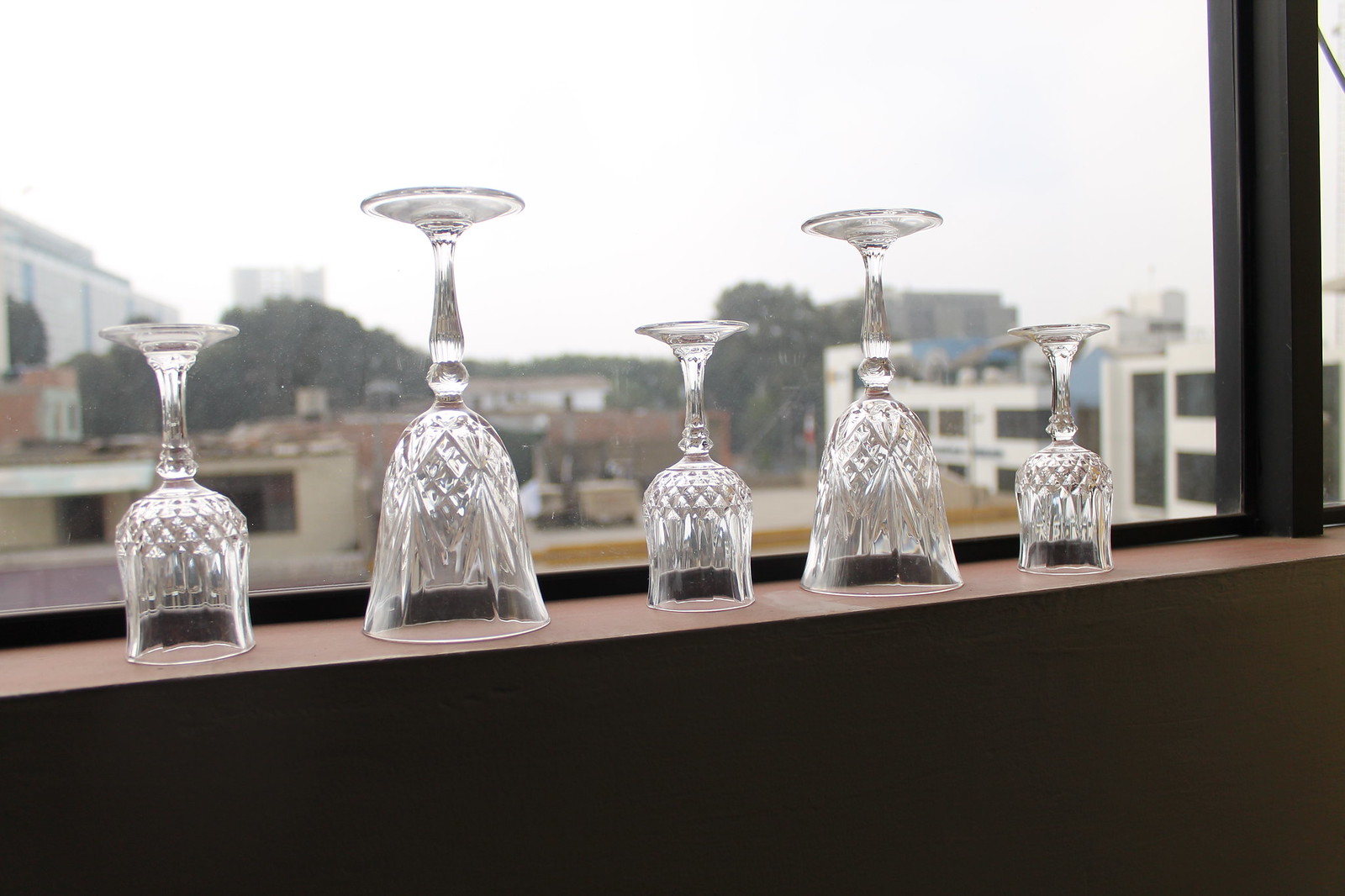A photograph captures a brown windowsill with five cut crystal goblets arranged upside down, creating a bell-like appearance with stems upward. The goblets are organized in a small, large, small, large, small pattern, where three are tulip-shaped likely intended for brandy, and two are more conical, suitable for wine, each adorned with a traditional honeycomb design toward the stem. The window, framed in charcoal gray or black, reveals an overcast sky making the exterior appear almost white. Beyond the window, blurred in the distance, are the white and brown architectural elements typical of a hospital or university campus, alongside large trees peeking over lower buildings, suggesting a serene but urban environment. The image is well-composed, with the foreground in sharp focus and the background softly blurred, emphasizing the elegant arrangement of the sparkling glasses on the sill.